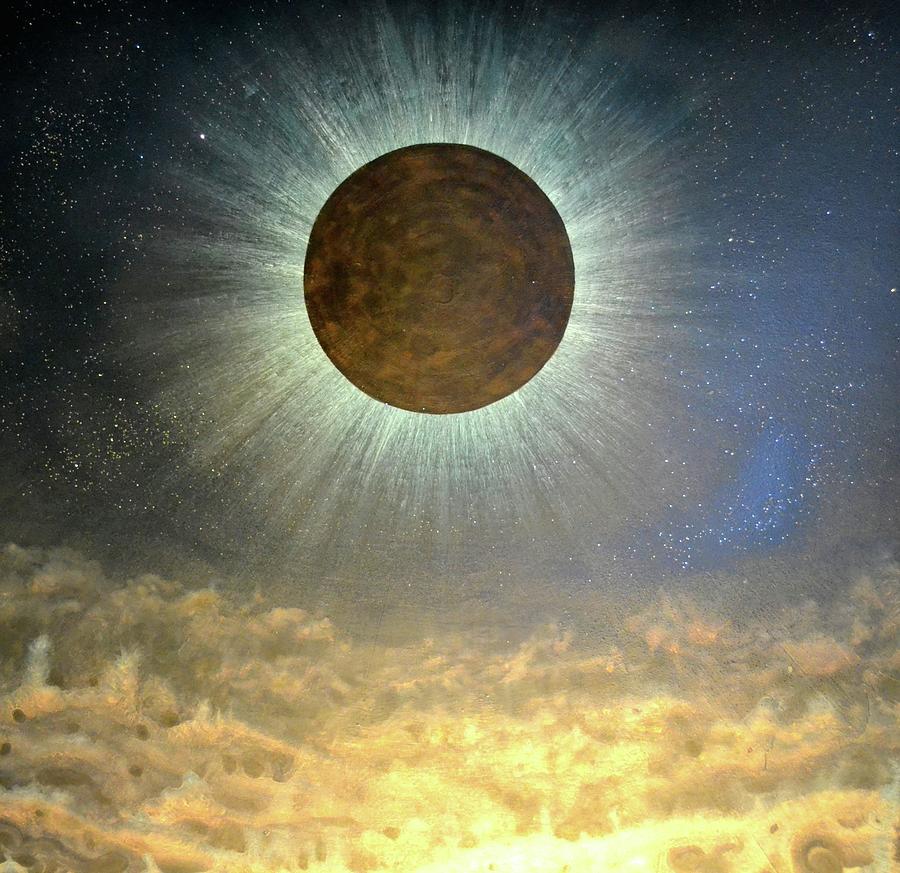The image appears to depict a dramatic and artistic representation of a solar eclipse. At the center top, a large, textured circle in varying shades of brown and black symbolizes the moon obscuring the sun. Radiating from behind this circle, you can see long, distinct sun rays piercing in different directions. The sky backdrop is divided into two segments: the left side is a deep black with numerous gray dots depicting stars, while the right side transitions into shades of blue, also speckled with white star-like dots. Towards the bottom of the image, a layer of brown-hued clouds or smoke envelopes the scene, with a hint of yellow sunlight breaking through at the center. The overall image has an appearance akin to a watercolor painting, capturing both the celestial event and the beauty of the surrounding sky.